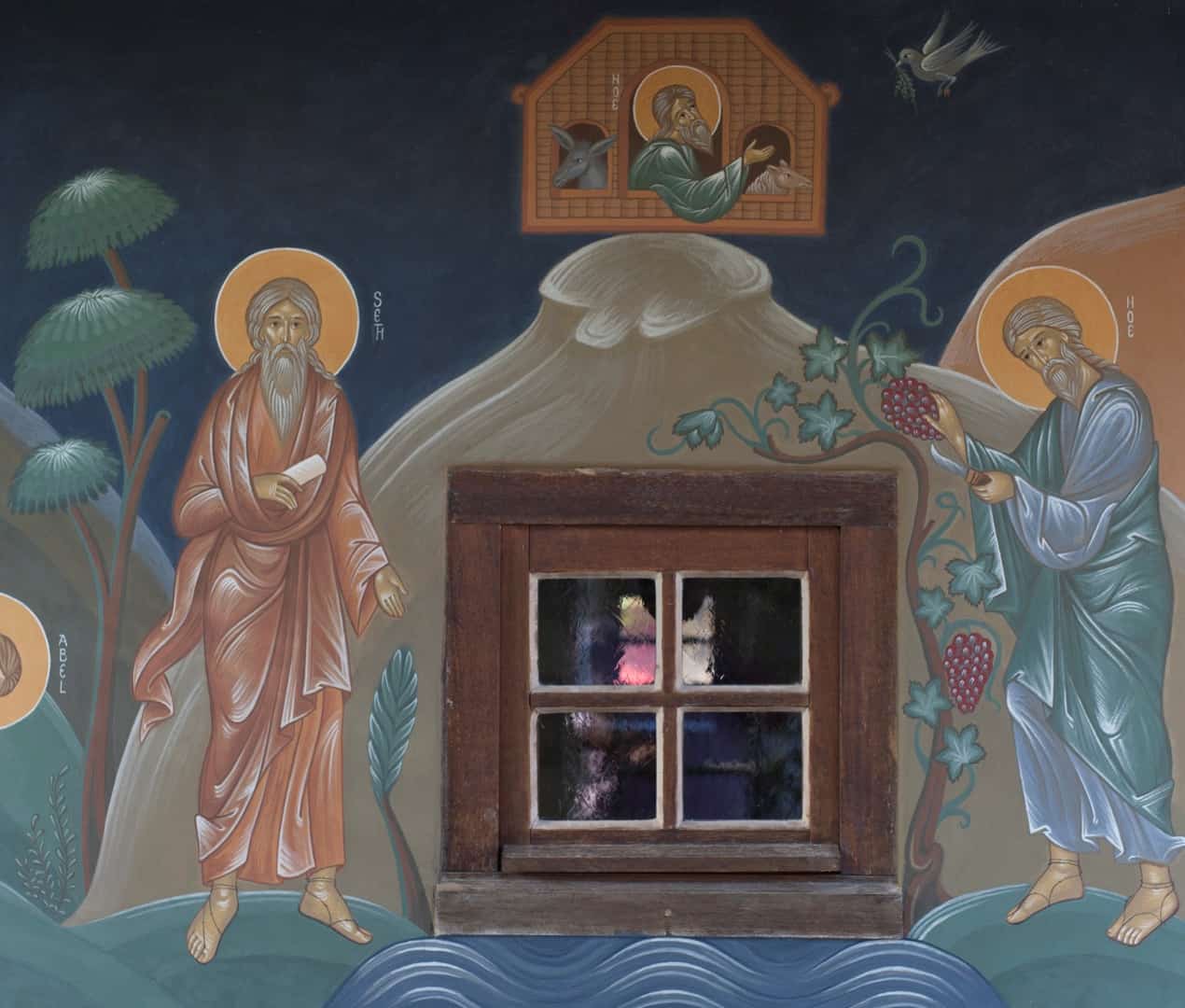This image appears to be an abstract rendition of a religious icon, possibly Eastern Catholic or Orthodox in style. It features three elderly, bearded holy men adorned with halos, each standing in a uniquely exaggerated and surreal landscape. 

On the left stands a man in robes of peach and orange hues, with a sun-like halo behind his head. On the right, another man wears blue and green robes, his halo matching the first's. This man appears much larger than life, nearly towering over an equally outsized window, from which he is picking large berries that dwarf the window itself. The scales of all elements are surreal and intentionally exaggerated, emphasizing the otherworldly and spiritual nature of the scene.

In the center of the image is an outlined, roughly sketched traditional home or barn with a oversized window showcasing hints of blue and pink. Above this structure, another man hangs out of a smaller window, wearing blue robes and also haloed. He is noticeably interacting with his environment, gazing towards a bird flying overhead with a branch in its beak. Beside him in the barn, two animals—possibly a sheep and a larger creature with prominent ears—are present, each hanging out of their respective windows.

The scene is set against a backdrop of stylized midnight blue sky, trees, and mountains, blending elements of nature into the abstract composition. Letters and words like "H-O-E," "S-E-H," and "A-B-E-L" are scattered randomly, adding to the enigmatic and mystical quality of this sketched artistic design.